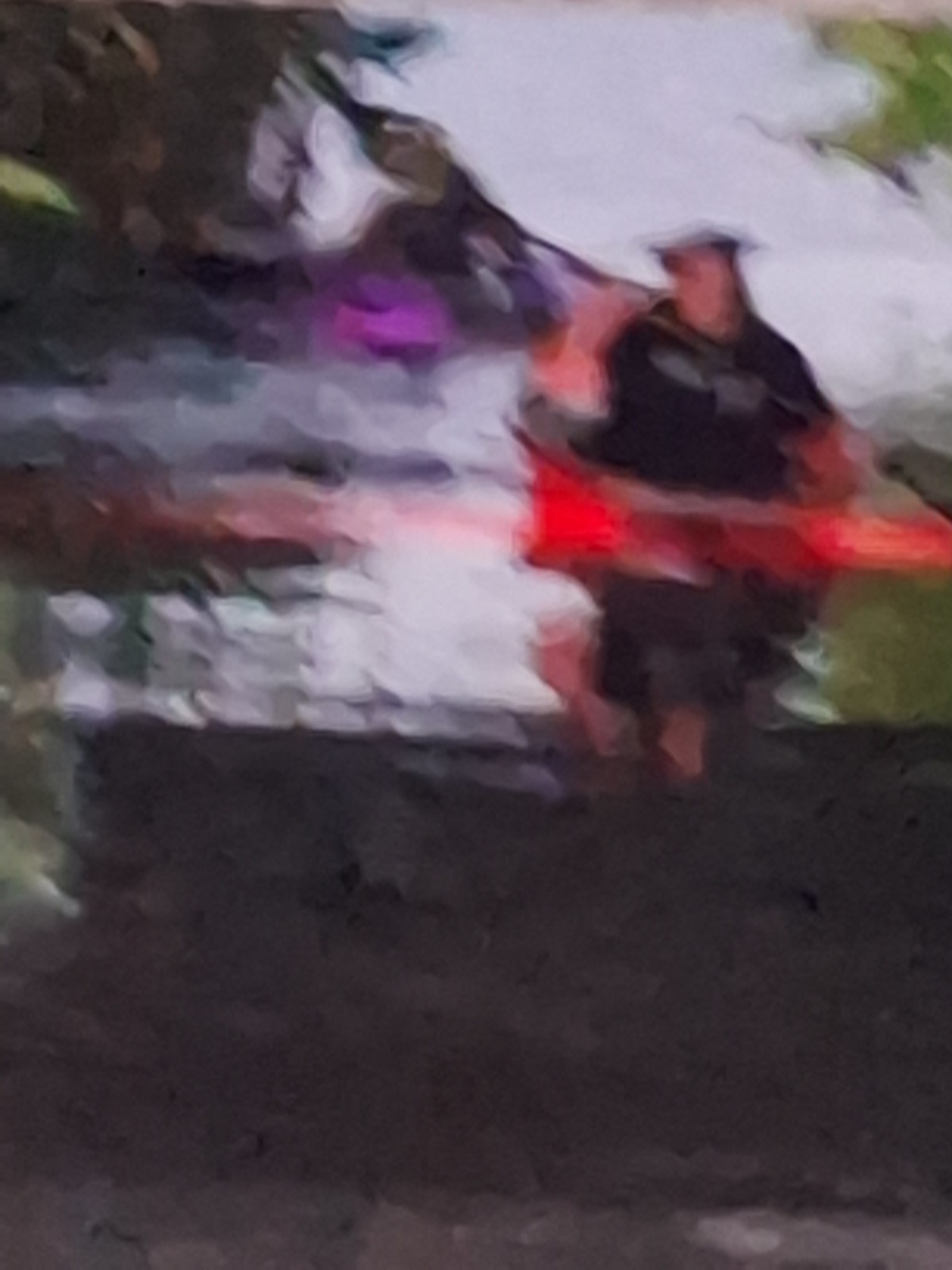In this image, a very blurry figure is positioned on the right-hand side, wearing a black t-shirt. Due to the blurriness, no distinct facial or bodily features are discernible. The bottom portion of the image is shaded in dark gray. The figure is standing vertically with a bright red object positioned in front of them. On the left side of the image, there is a series of light blue lights, followed by patches of black, pink, and blue colors. The upper left-hand corner features dark green hues, while the top right corner transitions to a light green. Between these green areas, light blue light shines through, possibly resembling the sky.